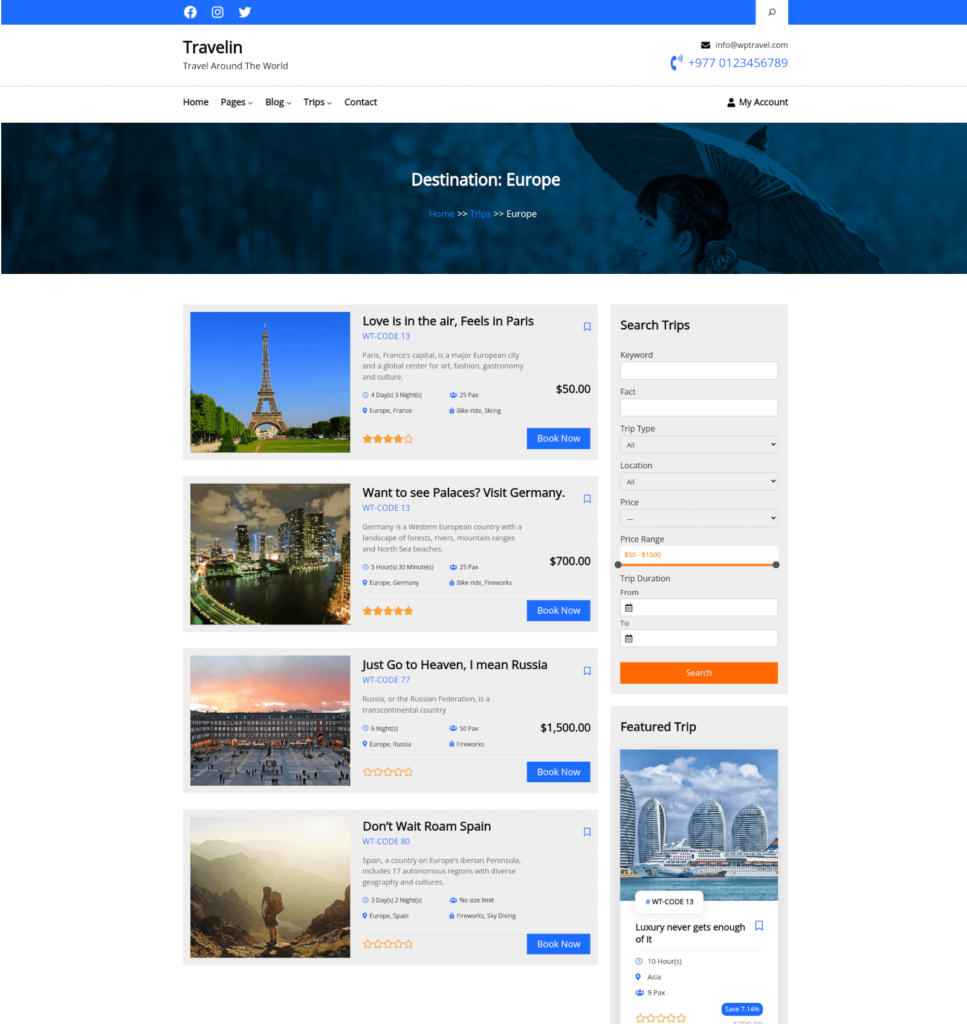This image shows a webpage from a travel booking website called "Travelin" (stylized as one word: "Travel-I-N"). The website prominently features a header with a big blue bar at the top that reads "Destination Europe." The navigation menu includes options such as Home, Pages, Blog, Trips, and Contact. 

Currently, the user has navigated to the "Trips" section, specifically viewing European travel options. Various travel packages are listed with the following descriptions and prices:

1. "Love in the Air: Feels in Paris" - priced at $50. This likely represents an excursion or activity, as the price is too low for accommodation.
2. "See Palaces: Visit Germany" - priced at $700.
3. "Just Go to Heaven, I mean Russia" - priced at $1,500.
4. "Don't Wait: Rome, Spain" - no price listed, urging users to "Book Now," suggesting a sense of urgency or exclusivity.

Additionally, there is a featured trip on the right side of the page with the tagline "Luxury: Never Gets Enough of It," though no price is provided for this particular offer.

This comprehensive layout provides a clear summary of European travel options, highlighting both budget-friendly and luxury experiences.